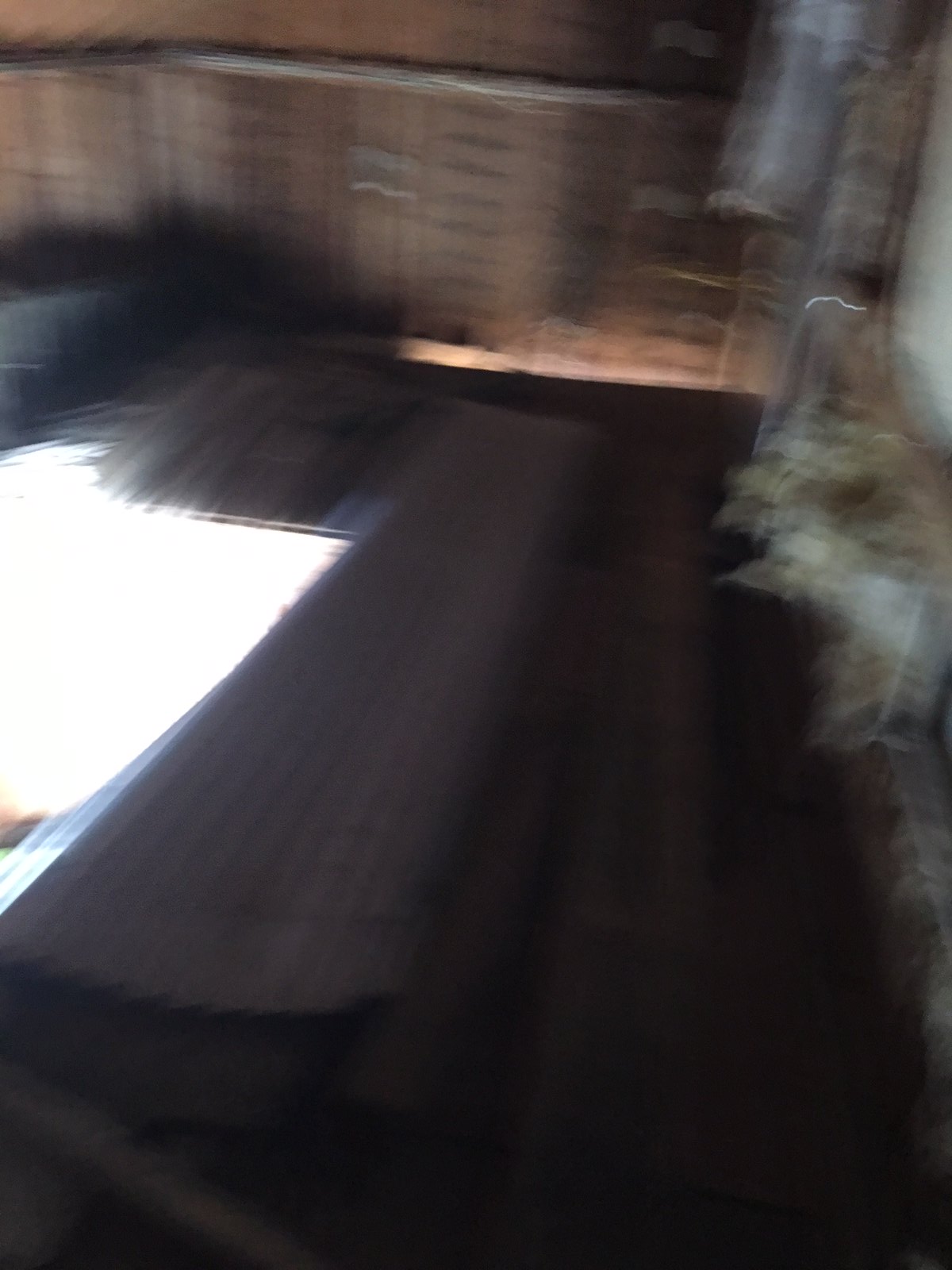The image presents a vertically rectangular frame, primarily shrouded in darkness and significantly blurred, suggesting an unclear focus or rapid movement. The setting appears to be an elevated level, likely the upper floor of a rustic barn, characterized by its raw, unfinished wood paneling that stretches upward within the frame. The wooden flooring, nearly black, adds to the overall dimness. Midway up the left side and extending towards the center, a bright white light penetrates the gloom, indicating the presence of a stairwell or opening through which natural light ascends from a lower level, providing a stark contrast to the surrounding environment.